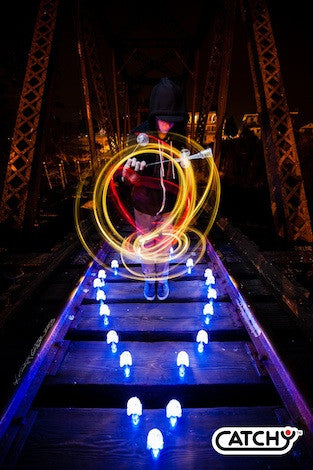In this captivating time-lapse photograph, a person stands on what appears to be a partially illuminated, possibly abandoned bridge or bridge-like structure with large metal supports resembling those found in suspension bridges. The individual, appearing steady amidst the dynamic scene, is dressed in a black hoodie with a white zipper and drawstrings, tan pants, and blue tennis shoes possibly resembling Vans. The person holds LED lights, which they whirl rapidly in circular motions, creating mesmerizing red and yellow light trails that dominate the image. Additional stationary lights on the wooden planks of the walkway, arranged in a teardrop or heart shape, add to the fantastical ambiance. Some of these surrounding lights resemble glowing mushrooms, further enhancing the scene’s surreal quality. The background reveals a faintly lit large structure or house, contributing to the mysterious and somewhat desolate atmosphere of the photograph.